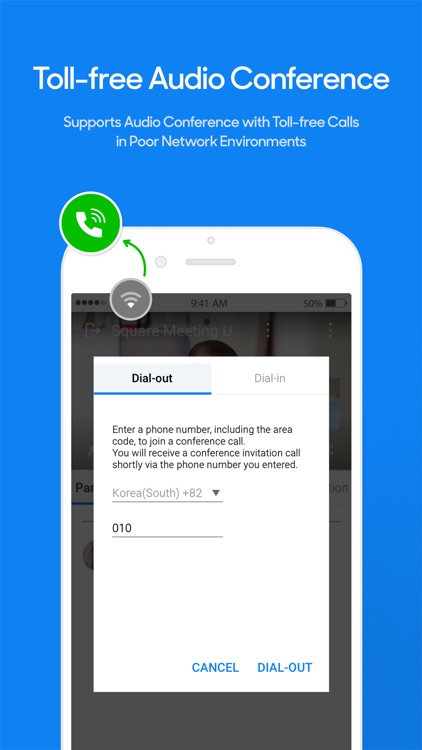In the image, the background is predominantly blue. Prominently displayed in white text are the words "Toll-free audio conference," explaining that the service supports audio conferencing with toll-free calls even in poor network environments. At the top of the image, there is a white smartphone featuring a camera and microphone. A large green circle emanates call waves from the handset, emphasizing the call functionality.

Additionally, the image includes a grey circle with the text "Lines," surrounded by smaller dots displaying the time "9:41 AM," the battery percentage "50%," and some other assorted details. The phrase "Swear I'm meeting you" appears alongside command buttons labeled "Dial out" and "Dial in."

Instructions are also visible, prompting the user to "Enter a phone number including the area code to join a conference call." It informs users that they will receive an invitation call shortly via the entered phone number. Another segment of grey text reads "Korea (South)" followed by the international dialing code "+82," and a dropdown menu showing "010." 

On the bottom right, options in blue text include "Cancel" and "Dial out." The edges of the screen, slightly out of focus, hint at the interface of a device or application, although details are obscured.